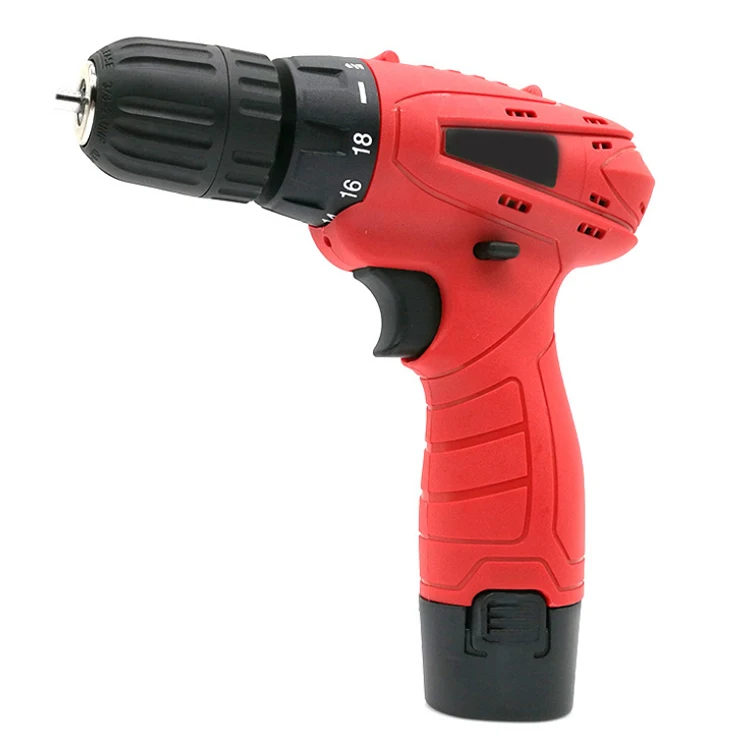This is a detailed product image of a rechargeable, battery-operated power drill on a plain white background. The drill stands upright on its black handle, with the drill bit piece facing left. The body of the drill is predominantly molded in a light, dull red plastic, with contrasting black elements including the trigger, a portion of the handle, and the base which houses the battery. At the front, the tip of the drill body is black with a silver bit. There is a round adjustable mechanism, marked with numbers 16 and 18, situated behind the drill bit. This mechanism allows the user to set the depth. The image highlights the simplicity and functionality of the drill, with its monochromatic color scheme of mostly red and black and minimalist white background providing a clear focus on the object itself.